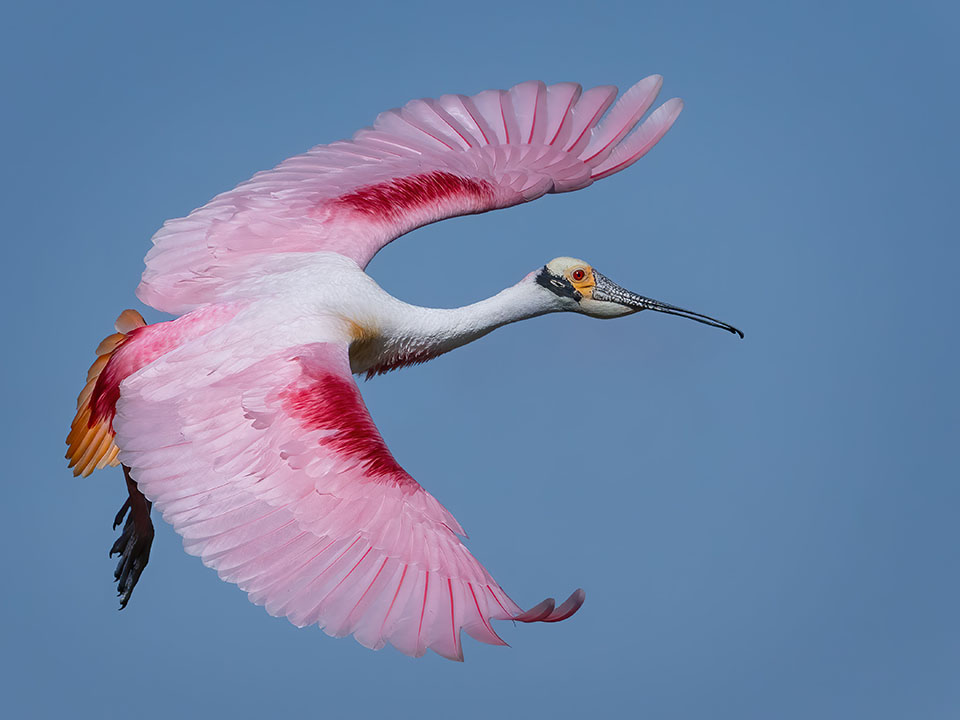The image depicts a vibrant ibis-like bird in mid-flight against a solid blue sky, indicating it was captured during a clear day. This stunning bird showcases an intricate color palette. The main body is predominantly white, with a narrow black beak that tapers to a point. Close to the head, there's a distinctive section of white feathers accentuated with an orangish patch around its eyes, giving it a striking appearance. Behind the head, a band of black feathers transitions seamlessly into the white feather base of the bird's body.

The wings are a vivid highlight, featuring dozens of spread-out, thin pink feathers, arranged in a graceful C pattern extending from the body. The mid-wing area exhibits a mixture of pink to red feathers, creating a textured, mottled effect. This transitions to almost transparently pink feathers towards the rear, with darker reddish hues near the tail. The tail itself has a more pinkish tone, interspersed with hints of orange.

The bird's black, webbed feet further emphasize its aquatic nature, an essential characteristic for a bird of this type. The image captures the bird with its wings uplifted, suggesting a motion frozen in time, adding to the dynamic beauty of this scene. The backdrop of a light blue sky without any clouds frames this exquisite creature perfectly, highlighting its vivid coloration and elegant form in flight.